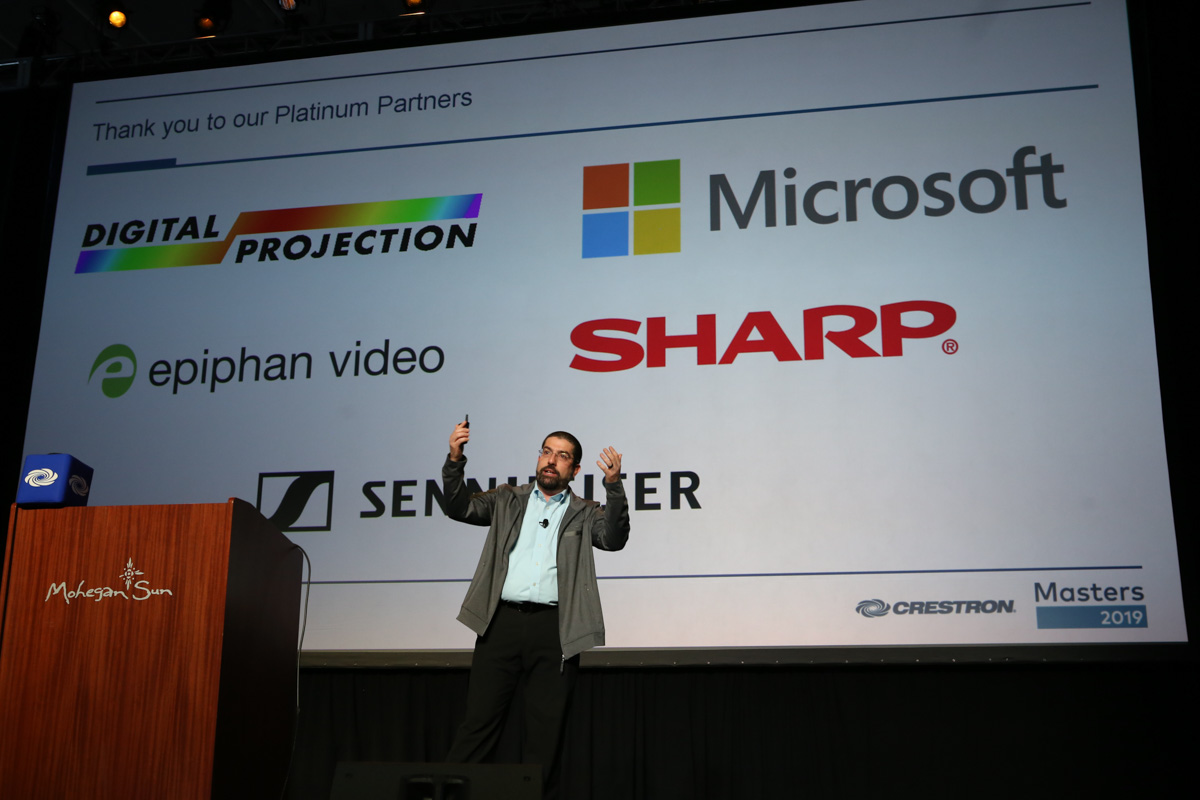In the image, a middle-aged, professional man is making a conference presentation on a stage, appearing smaller against the expansive background. He is wearing a light blue shirt under a green unzipped jacket or hoodie, paired with dark pants, and glasses with a full beard and short black hair. The man is enthusiastically gesturing with both hands raised, possibly holding a remote for a PowerPoint presentation in his left hand. 

He stands facing the audience, near a brown wood-grain podium emblazoned with "Mohegan Sun" and a sunburst logo, which also has a blue cube box with white swirls on top of it. Part of the backdrop behind him is a large white banner that notably reads, "Thank you to our platinum partners," showcasing the logos of several major companies such as Digital Projection, Microsoft, Epiphan Video, Sharp, and Sennheiser in their recognizable colors. Additionally, the banner includes the text "Crestron Masters 2019" located at the bottom right. A microphone is clipped to the center of his shirt, emphasizing his role as the speaker.